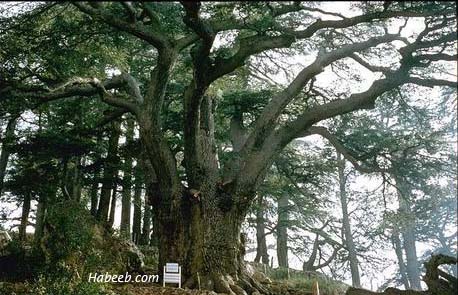This photograph captures a serene forest scene dominated by a massive tree slightly left of center. The tree boasts a thick trunk that splits into three large sections, sending out substantial branches that stretch into the upper left, top, and upper right sections of the frame, covered in lush foliage. Near the base, a white sign with unreadable text adds a touch of mystery, while a large rock adorned with vines sits nearby. Surrounding the main tree are thinner trees receding into the background, where snippets of a light blue or white sky peek through the canopy. At the bottom left of the frame is a watermark that reads "HABEEB.com," accompanied by a minimalist image of a chair, further emphasizing the untouched and tranquil nature of this forest scene without any human presence.